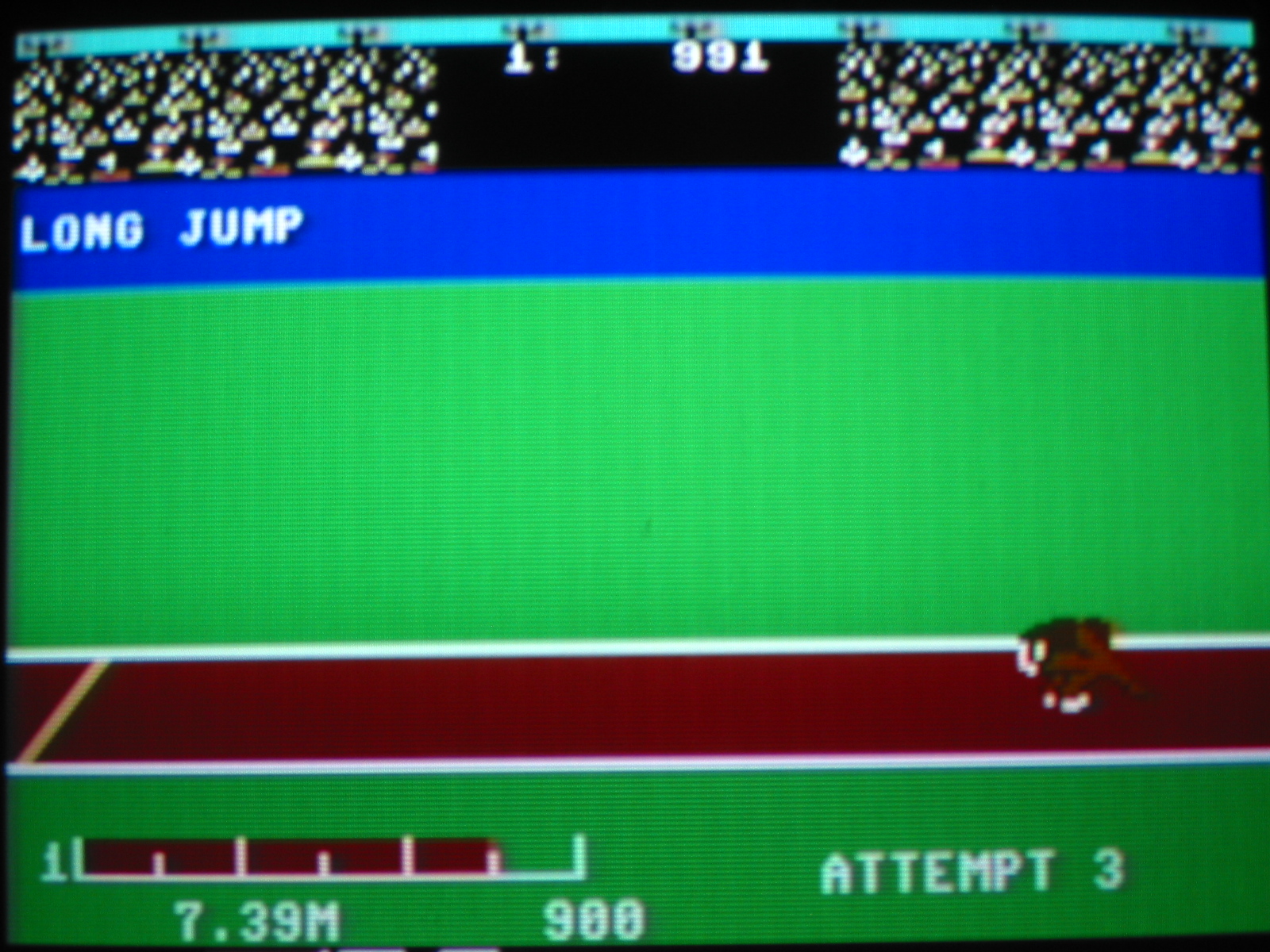The image appears to be a still from a video game depicting a long jump event, with various elements that make it visually engaging. In the upper left-hand corner of the screen, it prominently displays the words "LONG JUMP" in white, capital letters on a blue strip. This strip serves to label the event clearly for viewers. Beneath the strip, there are numerous small dots that represent a large, indistinct crowd of spectators, giving the scene a lively atmosphere.

The mid to lower right-hand portion of the image shows a character who has just completed their jump. The character, a small sprite that looks like a bird or a round creature, is positioned with bent knees in front of their feet, suggesting the landing phase of the jump. The long jump track itself is a dark brown or burgundy rectangle with white outlines and a line marking the jump point. Surrounding the track is a green area that resembles a field, adding to the sports setting.

At the very bottom of the screen, the image displays a measurement gauge labeled from 1 to 900 meters, which reads "7.39 M," indicating the distance of the jump. This gauge is accompanied by the text "Attempt 3," highlighting that this was the character's third jump attempt. Additionally, elements of the image include a green wall behind the track and a blue banner above it, further enriching the scene with complementary background details. The overall style of the image conveys a pixelated, video game aesthetic.

Combining these elements, the detailed caption is:

A still image from a video game captures the moment just after a long jump event. In the upper left corner, the words "LONG JUMP" are prominently displayed in white, capital letters on a blue strip. Below this, a mass of small dots represents a lively crowd of spectators. The mid to lower right portion shows a character, resembling a small sprite or bird, bent over just after landing. The long jump track, a dark brown or burgundy rectangle with white outlines, is set against a green field. At the bottom of the screen, a measurement gauge from 1 to 900 meters reads "7.39 M," marking the distance of the jump, along with the text "Attempt 3," indicating the third attempt. Background elements include a green wall and a blue banner, enhancing the sports event atmosphere with a pixelated, video game aesthetic.